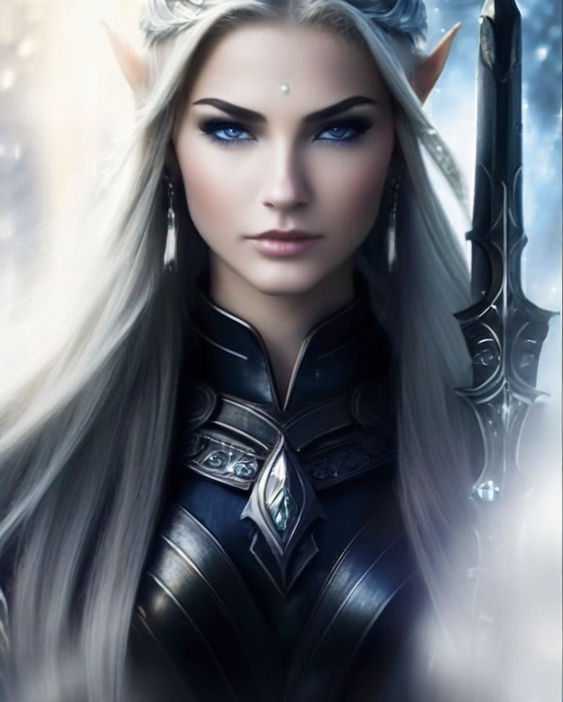This digital illustration depicts a female elf warrior with fantastical attributes. She has long, silver-white hair styled in a half-updo, which cascades around her pointed, elven ears. Her striking blue eyes and slightly blushed cheeks frame her defined features, including dark eyebrows and an intense, determined expression. Adorning her ears are long, elegant earrings.

Clad in a regal, dark blue and metallic-grey armor, she stands ready for battle. The armor is intricately designed, featuring a leaf-shaped emerald below the neckline. In her right hand, she wields a long iron sword embellished with embedded jewels. Adding to her mystical appearance, she has horns emerging from her head. 

The background of the image is hazy and wispy, creating an ethereal atmosphere, with hints of a starry night sky peeking through. This vertical illustration focuses primarily on the warrior, making her the striking centerpiece of this anime-inspired artwork.